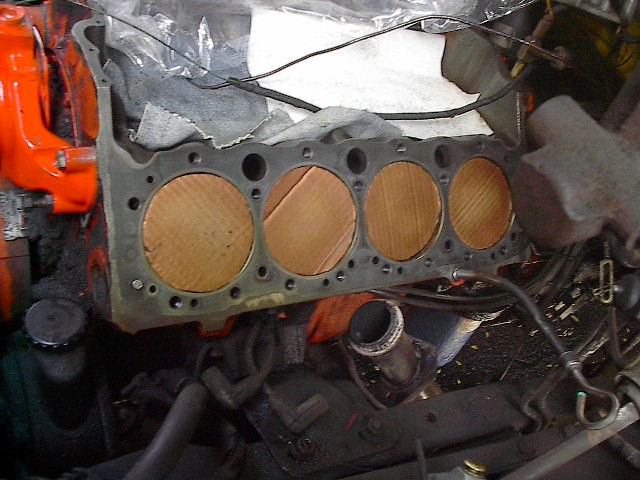A highly detailed color photograph captures the intricate internal components of a large truck engine or possibly a car engine. The image is taken from within the engine compartment, featuring a dark perimeter which draws focus toward the detailed center. Prominently, a bright industrial orange, curved metallic structure occupies the upper left quadrant, while a network of dark wires crisscrosses a central white section. Below and to the right of this, black spark plug wires are visible, partially overlaid by a gray steel strip featuring four large, evenly spaced circular cutouts along its length, accompanied by smaller holes designed for screws or fasteners. Behind this strip, a layer of tan cardboard is discernible. Additional engine components such as various valves, cords, and a possible silver hook or metal rod populate the scene, adding to the mechanical complexity. Scattered around, there are also hints of light blue material and white paper, suggesting packaging or insulation materials amidst the functional parts, along with a section that could serve for oil or water input.